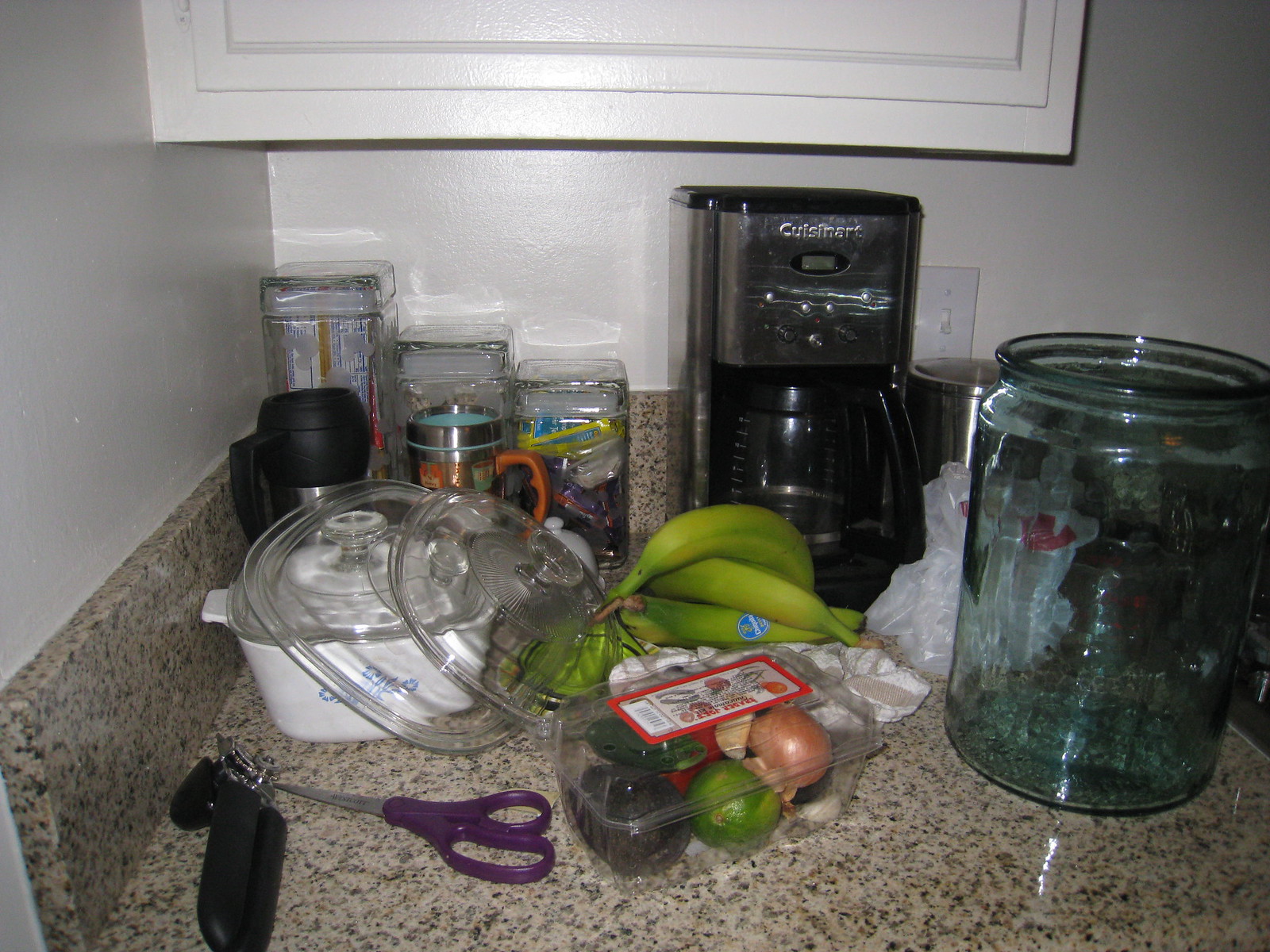This photograph captures a section of a kitchen counter made of stone, featuring a matching stone skirting that outlines its edges. Above the counter, a pristine white cupboard provides a backdrop. The counter itself is adorned with various kitchen essentials: a filter coffee maker prominently placed, with a cluster of green bananas resting in front of it. An empty glass jar without a lid stands next to a pair of kitchen scissors with distinctive purple handles. A clear plastic container brimming with an assortment of fruits and vegetables adds a touch of color. Additionally, a white pot with a glass lid is visible, along with two thermal containers shaped like cups. Completing the scene are three square-shaped glass jars that are filled with different food items, meticulously arranged in a row.